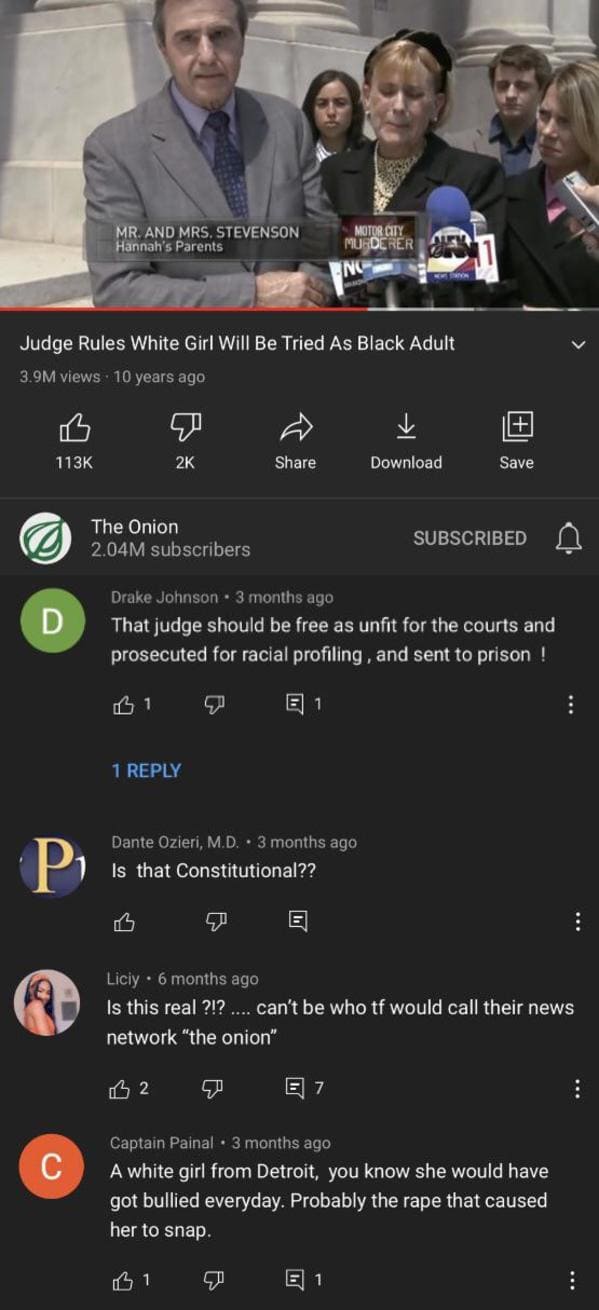Here's the cleaned-up and detailed caption for the image:

---

The image is a rectangular box oriented vertically, captured from a social media platform, possibly YouTube. At the top of the image, there is a photograph featuring a group of five individuals, including Mr. and Mrs. Stevenson, identified as Hannah's parents, alongside others at a press conference. Microphones are clearly visible in front of them, suggesting they are addressing the media.

Below the photograph, the rest of the image has a black background with white text that reads: "Judge Rules White Girl Would Be Tried as Black Adult." This video has amassed 3.9 million views over the span of 10 years.

Overlaying the image are several interactive icons including 'thumb up,' 'thumb down,' 'share,' 'download,' and 'save.' Indicators show that the channel, identified as "The Onion" with 2.04 million subscribers, is subscribed to by the person viewing this video.

Below the video, the comments section reveals a variety of reactions:
- One comment critiques the judgment, stating: "Judge should be free as unfit for the courts and prosecuted for racial profiling and sent to prison."
- Another user questions the legality: "Is that constitutional?"
- A third expresses skepticism: "Is that real? Can't be. Who the fuck would call their news network 'The Onion?'"
- Yet another comment provides a personal reflection: "A white girl from Detroit? You know she would have got bullied every day. Probably the rape that caused her to snap."

The collection of comments adds layers of complexity and public opinion to the controversial headline depicted in the video.

---